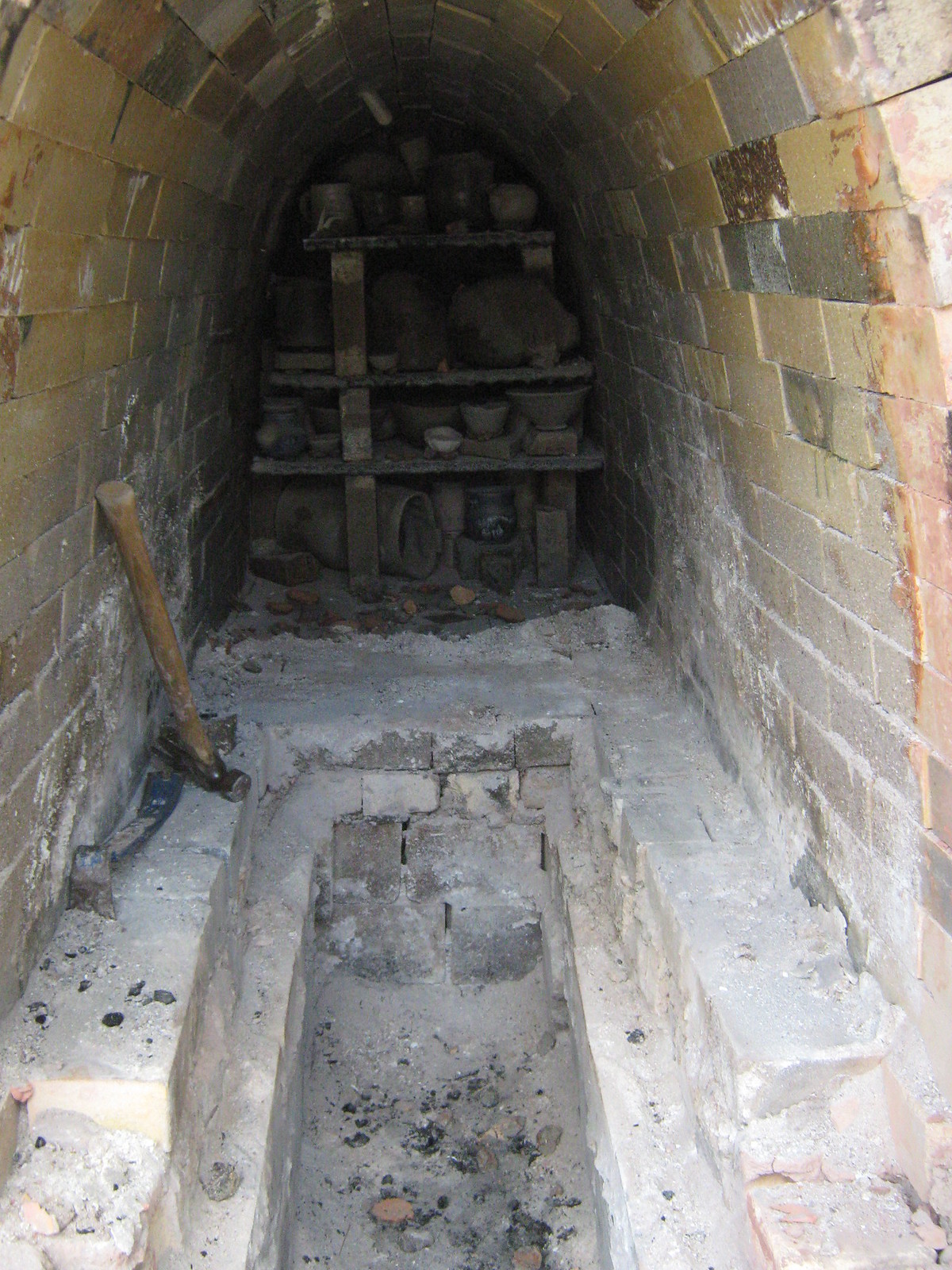This photograph captures the interior of an ancient, tomb-like structure with a distinctly domed, arched shape created from a mosaic of bricks in varying shades of brown, gray, and occasionally black. The space is dimly lit, emphasizing the age and secrecy of the site. Dominating the center of the room is a rectangular pit, which narrows as it descends and has traces of red and black substances at its base, suggesting the remains of previous activity.

To the left of the pit, a pair of excavation tools—a sledgehammer with a brown handle and a metal crowbar—lie against the old brick walls, indicative of ongoing or prior archaeological digging. Alongside the back wall, there are shelves constructed from aged wood, displaying an array of pottery, including bowls and vases in earthy tones. The ground and lower walls are dusted with a light gray ash, adding to the atmosphere of antiquity and long-abandoned use. The photograph lacks any textual clues, leaving its exact origin and purpose open to interpretation, though it evokes the sense of an archaeological discovery possibly deep within an ancient pyramid or tomb.